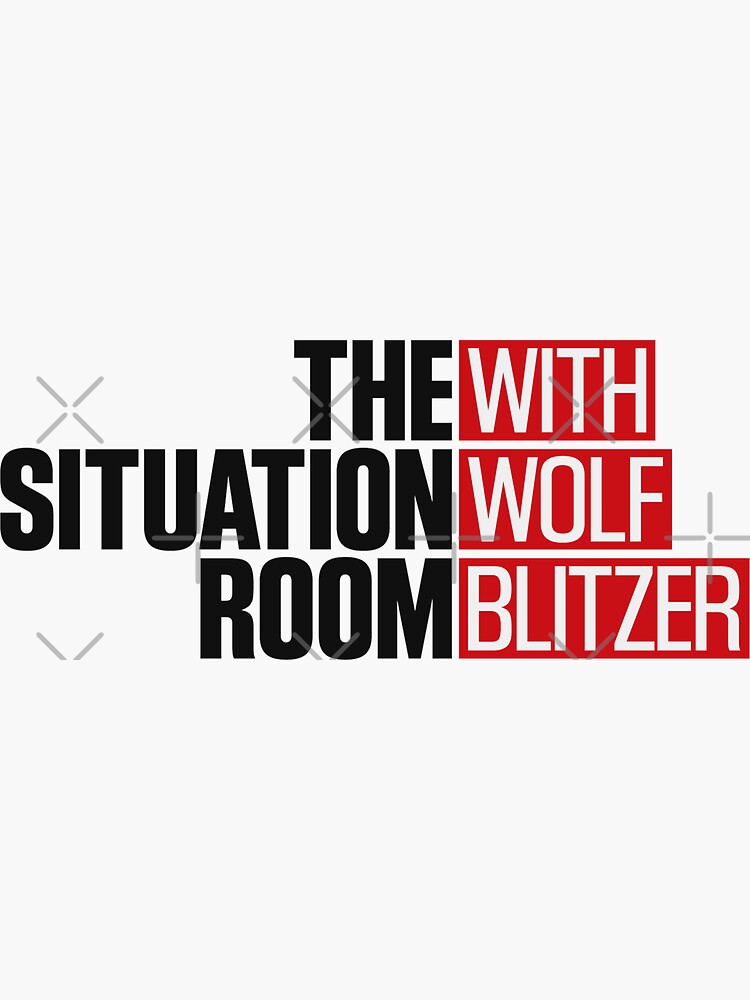The image is a vertically-oriented white rectangle serving as an advertisement for a TV show called "The Situation Room with Wolf Blitzer." The text is prominently featured in the center of the image. "The Situation Room" is written in bold, black, capital letters stacked vertically. To the right, "With Wolf Blitzer" appears in white, capital letters enclosed within red rectangular boxes. The entire image is watermarked with gray X and plus sign patterns, indicating it is copyrighted. There are no other elements such as people or animals, making the text the focal point.